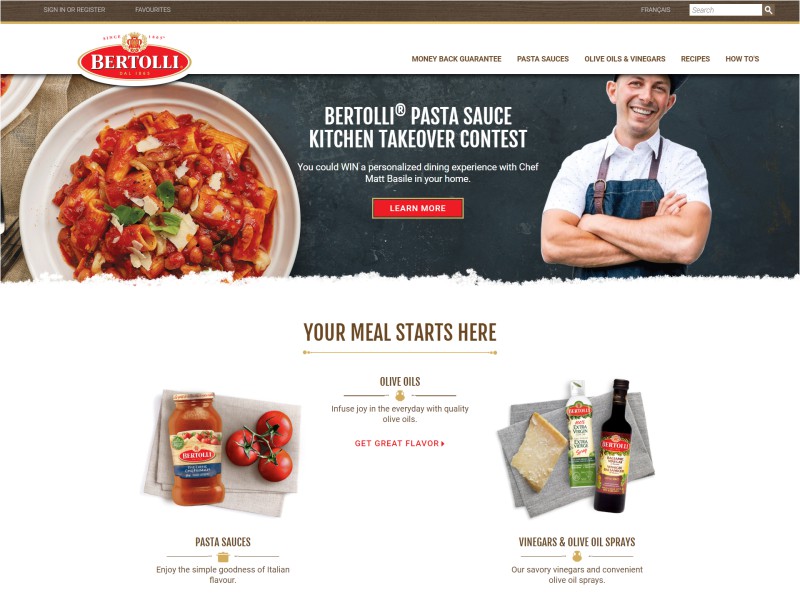A screenshot of Bertolli's website features a small brown bar at the top with a search bar labeled "Search" and a white magnifying glass icon in the top right-hand corner. Below this, the background turns white, displaying the Bertolli logo, which consists of a red oval with "Bertolli" written in the center and a small emblem embossed at the top.

To the right of the logo are navigation options including "Money Back Guarantee," "Pasta Sauce," "Olive Oils and Vinegars," "Recipes," and "How-Tos." Beneath this, the background image changes to gray, showcasing a smiling man with crossed arms wearing overalls. The text next to him reads, "Bertolli Pasta Sauce Kitchen Takeover Contest," asking, "Could you win a personalized dining experience with Chef Matt Bazile in your home?" Below this promotional text is a red "Learn More" button.

To the left, there is an image of a plate of rigatoni pasta. Underneath it, the text reads, "Your meal starts here, olive oils. Infuse joy in every day with quality olive oils, get great flavor." To the left of this, another section mentions "Pasta Sauces," with the tagline, "Enjoy simple goodness of Italian flavor." On the right, the caption says "Vinegars and Olive Oil Sprays," describing the products as "Our savory vinegars and convenient olive oil sprays." Images of the pasta sauce and olive oil spray products are also displayed.